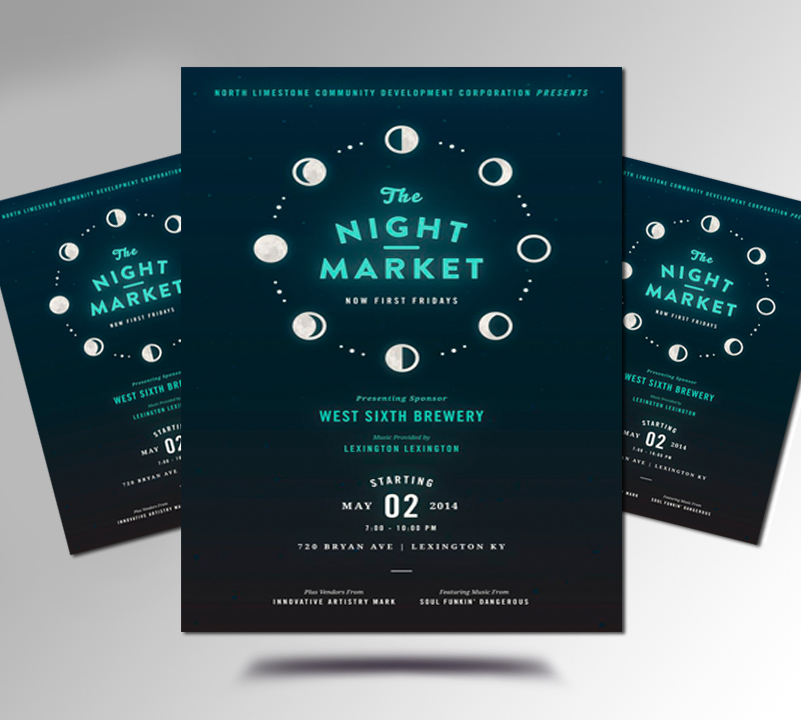The image is an invitation or advertisement featuring a dark blue, almost black, background with green and cyan-colored text. The main poster is prominently displayed in the center with two identical, smaller posters fanned out to the right and left. At the top, in cyan text, it reads, "North Limestone Community Development Corporation Presents." Below this is a circular arrangement of the phases of the moon, depicted in white. Inside this circle is the bold, cyan text, "The Night Market, Now First Fridays." Further details in green text include "Presenting Sponsor, West 6th Brewery, Music Provided by Lexington Lexington," along with the event starting details, "Starting May 2, 2014, 7 to 10 p.m., 720 Bryan Avenue, Lexington, Kentucky." Additional information mentions vendors like Innovative Artistry and Mark, with musical performances by Soul Something and Dangerous.